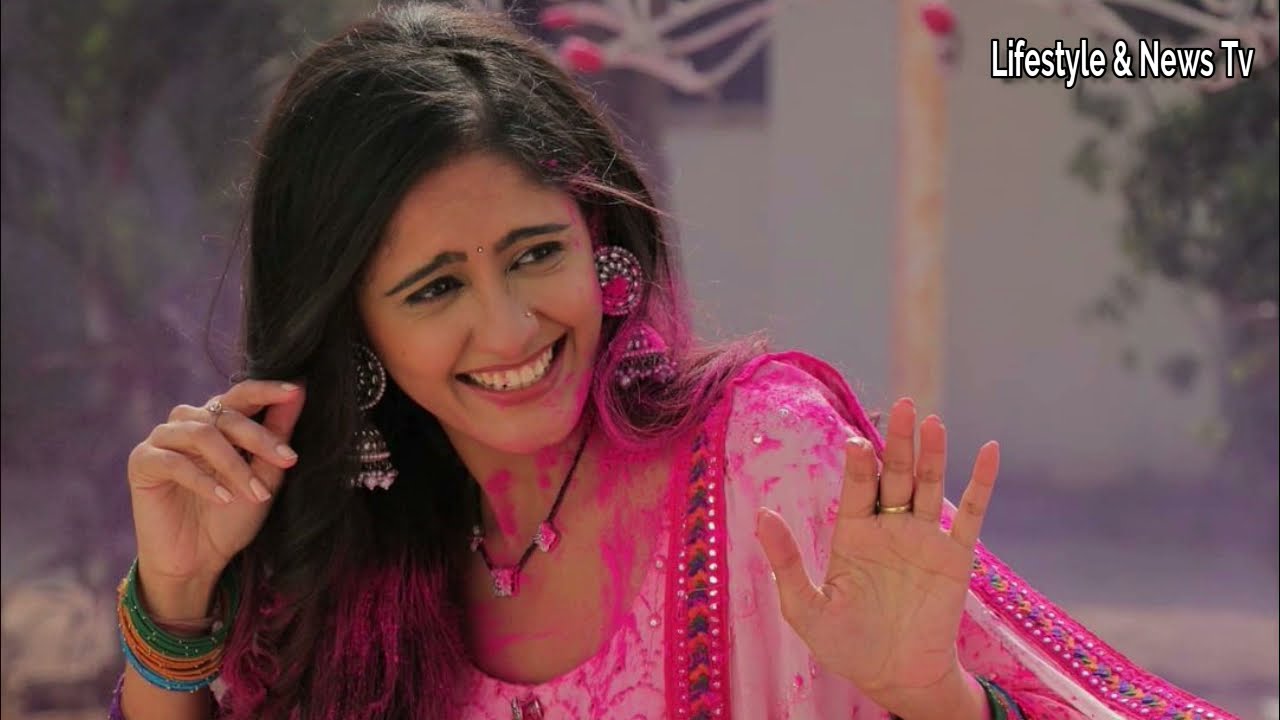The image features Indian actress and lawyer Ayesha Singh, adorned in a vibrant, traditional Indian outfit with a pinkish hue, detailed stitching, and dark pink blotches. Her dark black hair cascades beneath her left shoulder, framing a smiling face that slightly looks to the right. Her expression is a mix of playful and perhaps slightly surprised, with her mouth open, revealing her teeth. She is adorned with numerous accessories, including large, ornate round earrings, one of which has pink paint on it, a decorative nose ring, and a gem-adorned bindi between her eyebrows. Her hands are held up as if gesturing or waving; both middle fingers showcase rings, and the left hand is decorated with colorful bracelets in green, orange, and blue. Pink paint is also visible on her neck and face, reminiscent of festivities such as Holi, the Festival of Colors in India. The background is a soft blue-gray, slightly out of focus, giving prominence to Ayesha's exuberant presence. In the upper right corner of the image, white text reads "Lifestyle and News TV."